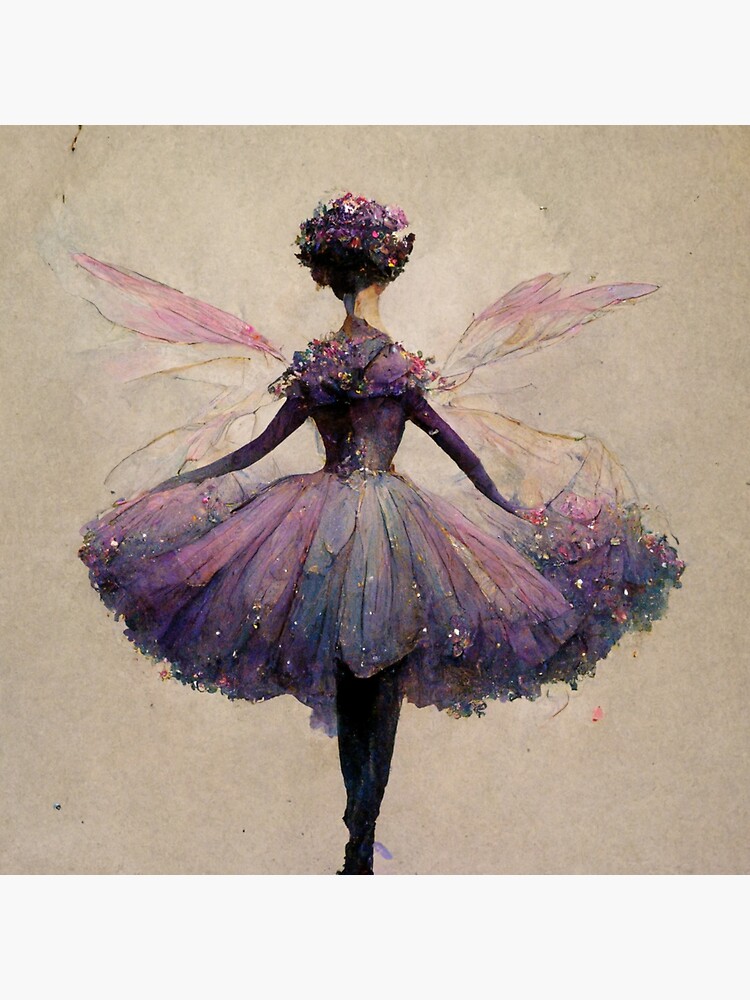The image depicts a delicate watercolor painting of a child-like ballerina with fairy wings, captured from behind. The ethereal figure is adorned in a sparkling purple tutu dotted with white highlights, flaring out to knee length, complementing her dark tights and matching long-sleeved top. Her ensemble is striking against the nuanced background of soft pinks, blues, and grays, which darken towards the edges and corners, creating a vignette effect. A shell-like collar draped over her slender neck is adorned with purple, pink, and white flowers, blending seamlessly with her dark hair. The fairy-like ballerina’s wings are a harmonious mix of white and pink hues, adding to the whimsical nature of the scene, enriched with subtle glitters that catch the light and add a touch of magic to the setting.